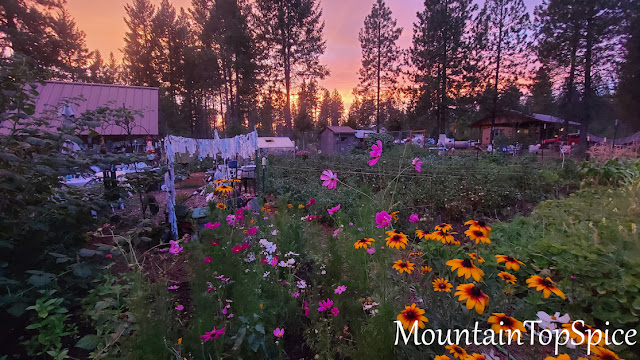The photograph depicts a picturesque homestead nestled in the countryside, dominated by a serene landscape of tall evergreen trees in the background. At the forefront, a sprawling garden teems with lush greenery and vibrant flowers—pink, white, yellow, and orange, with some daisies and peonies. The garden entrance is festively adorned with shredded fabric. Several cabin-like outbuildings and structures are scattered throughout the scene, including one with a red vehicle, possibly a Jeep, parked beside it. Multiple cars are parked around the area. White clothes hang to dry on a clothesline. The sky exhibits a gradient from orange to light blue, suggesting either dawn or dusk. The image is marked with the watermark "Mountain Top Spice" at the bottom.